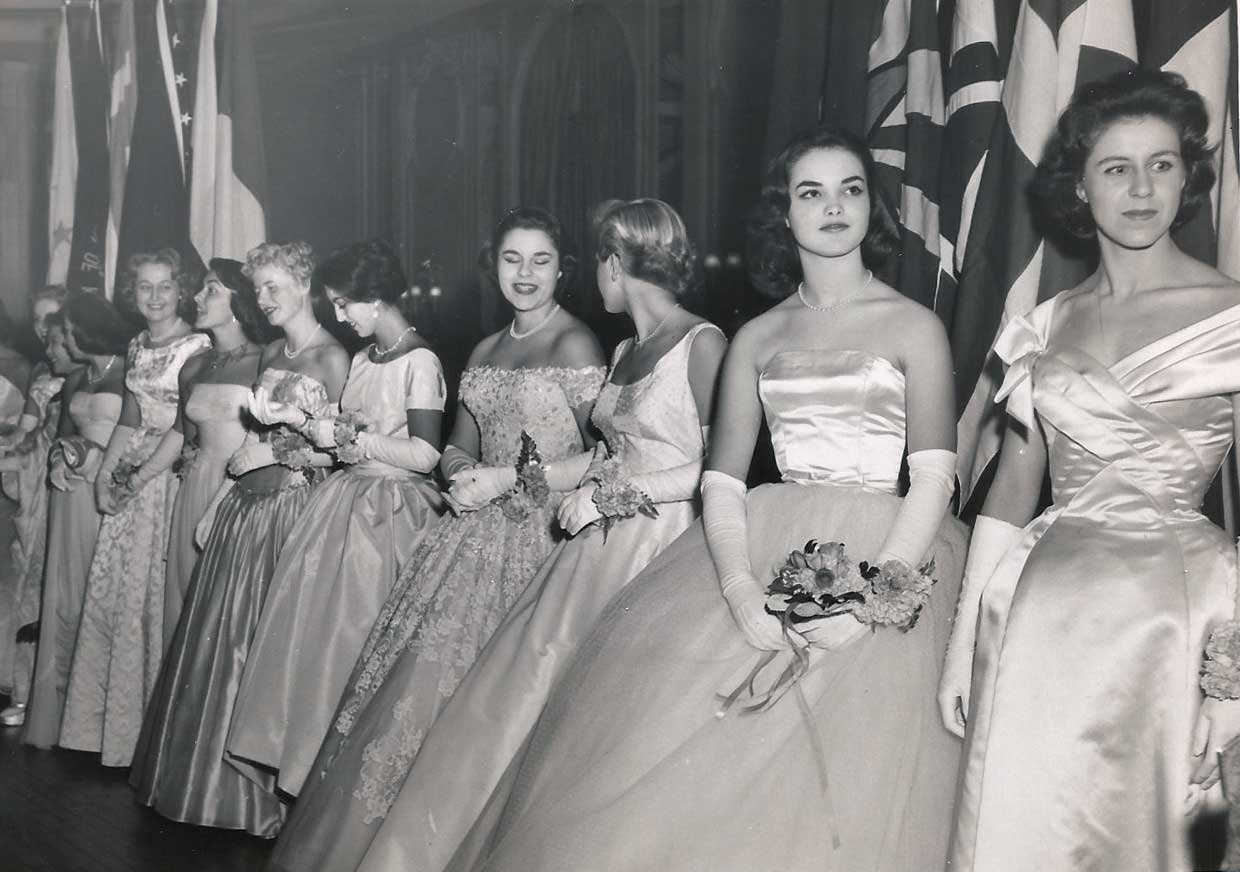This is an old, black-and-white photograph depicting approximately 11 to 15 young women standing in a horizontal line, possibly from the 1960s based on their hairstyles. They are all dressed formally in satin wedding dresses with long white gloves and necklaces, some of which are draped off their shoulders. Most of the women are holding bouquets of flowers, with some wearing flowers around their wrists. The setting appears to be formal, possibly within a cathedral-like venue, as suggested by the large brown wall with arch cutouts and the visible doors in the background. The women are engaged in various postures: some are conversing and laughing, while others are looking at their flowers or gazing around. In the top corners of the image, numerous flags are bunched together, obscuring their details. The floor beneath them seems to be wooden, and a curtain can be seen behind the group. The overall scene exudes a celebratory and elegant ambiance.